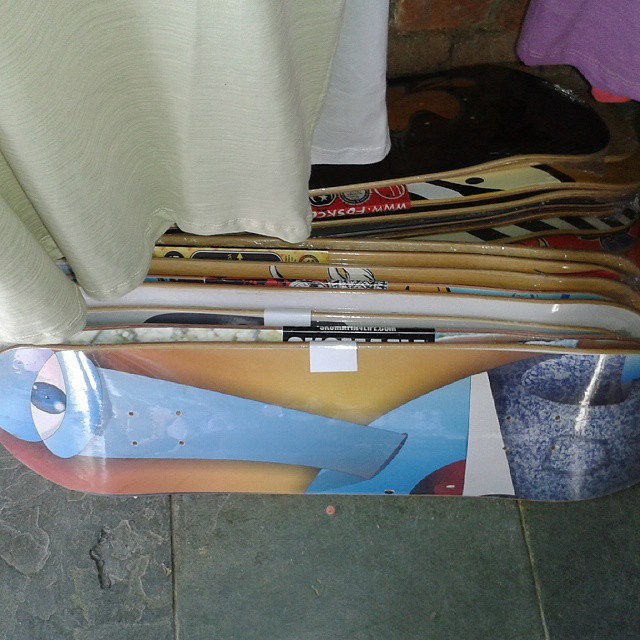This indoor color photograph captures a stack of approximately a dozen skateboard decks, notably without wheels, positioned upright on their long sides in a disorganized pile on a gray slate-like tiled floor. The floor appears dirty and the tile on the far left is notably damaged, with a deep indention suggesting something heavy was dropped on it. The skateboards exhibit a range of vibrant patterns and colors, though many are wrapped in plastic, obscuring some details. Most prominent is a skateboard with a striking design featuring an eye with yellow ovals on a blue background. Another deck showcases a red label. The backdrop includes a brownish brick wall and parts of a beige and white curtain on the left side, with a purple fabric, possibly part of a garment, visible on the upper right edge. The image's cluttered and casual arrangement, alongside the presence of various draperies, suggests the photo was taken in a somewhat untidy, perhaps residential setting.